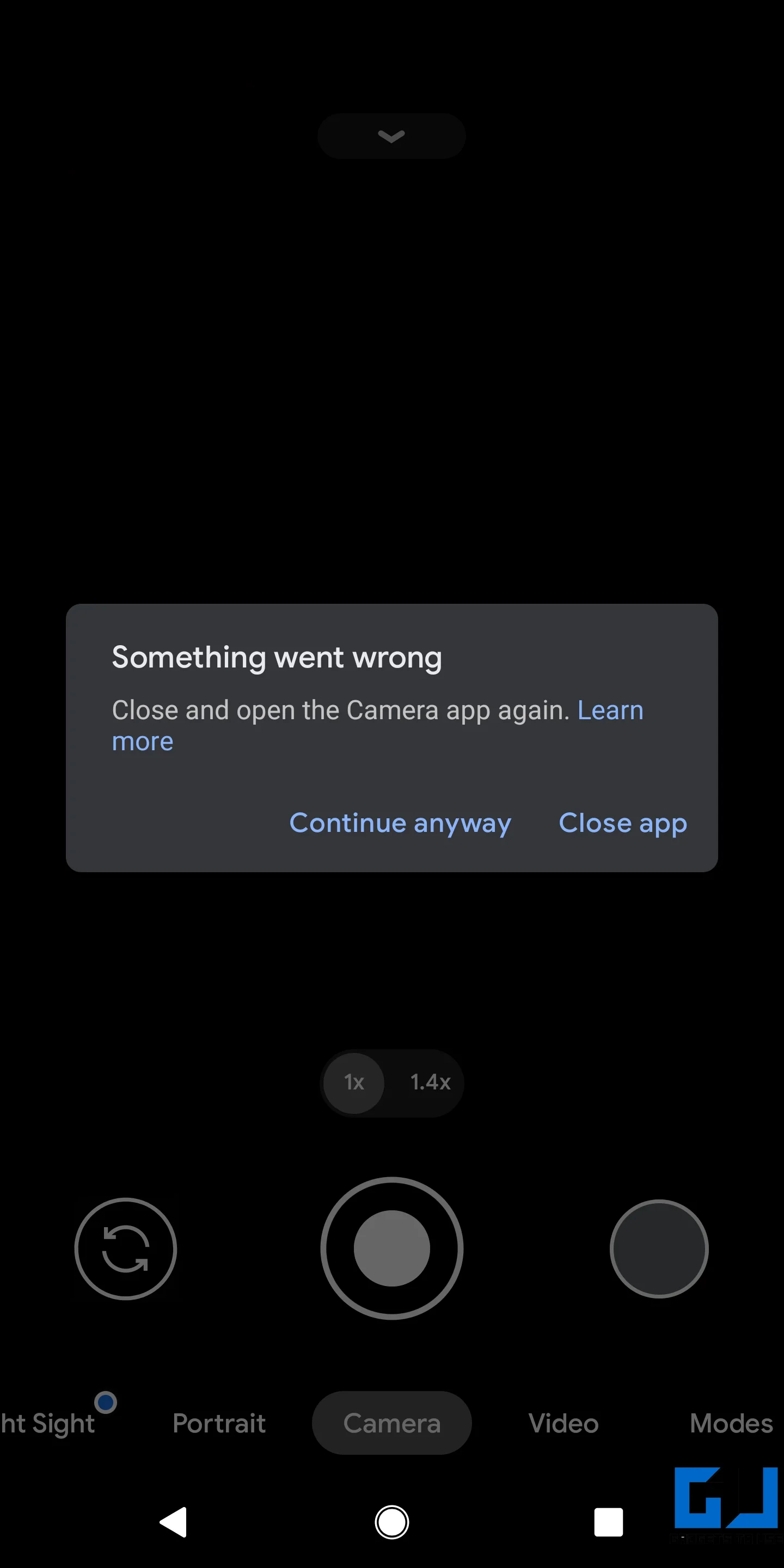A vertical rectangular screenshot of a smartphone interface with a black background shows a grayed-out downward-pointing arrow in a small tab at the top. Centrally placed is a light gray notification area with white text stating, "Something went wrong. Close and open the camera app again." Below this message, there is a clickable blue hyperlink saying “Learn more.” At the bottom of this gray notification area, there are three blue text options: "Continue anyway," "Close app," and a two-directional arrow symbol in a circular design.

Below this notification, there is a slider control for zoom, displayed as "1x" on the left and "1.4x" on the right, with a light gray circle currently toggled to "1x." 

The camera interface itself has a few symbols: a central circular button with a gray outline and a filled gray dot, flanked by a two-directional circular arrow icon on the left and a light-bordered dark gray circle on the right. 

Further down, a menu bar is visible with several options: "Sight" in gray with a blue dot encircled in gray near the top right of the "T", "Portrait," "Camera" highlighted in an elongated gray oval, "Video," and "Modes."

At the very bottom, the interface has three navigation icons: a triangle pointing left for 'back,' a circle, and a square for various navigation functions. The blue letters “GJ” appear at the bottom right. This screenshot indicates that there are issues with accessing or using the camera app on the device.